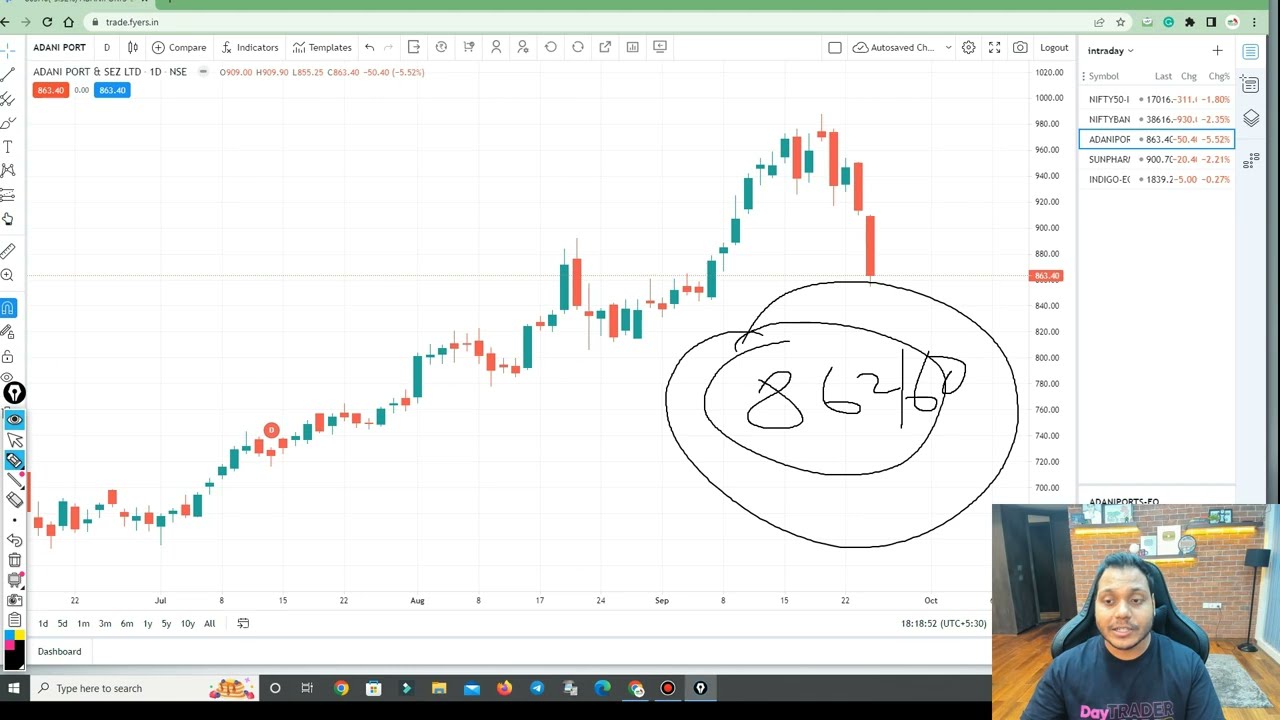The image is a detailed screenshot from a computer screen, likely during a live stream on platforms like Twitch or YouTube, showcasing a session of stock trading. The main part of the screen features a Windows 10 desktop capturing a detailed candlestick chart of AdaniPort Limited, with stock trends depicted in green and red bars indicating upward and downward trajectories, respectively. A significant price point, 86460, is circled twice sloppily in the middle of the chart, indicating the trader's targeted price or key interest level. In the bottom right corner, a webcam view shows a young man with dark skin, black hair, and wearing a black shirt with pink text saying "Day Trader." He is seated in a high-backed gaming chair, set against a backdrop of a brick wall, hardwood floors, a gray carpet, a black lamp, and shelving. The Windows 10 taskbar is visible at the bottom of the screen, along with various icons and a browser window's top bar with a light green hue and navigation buttons.